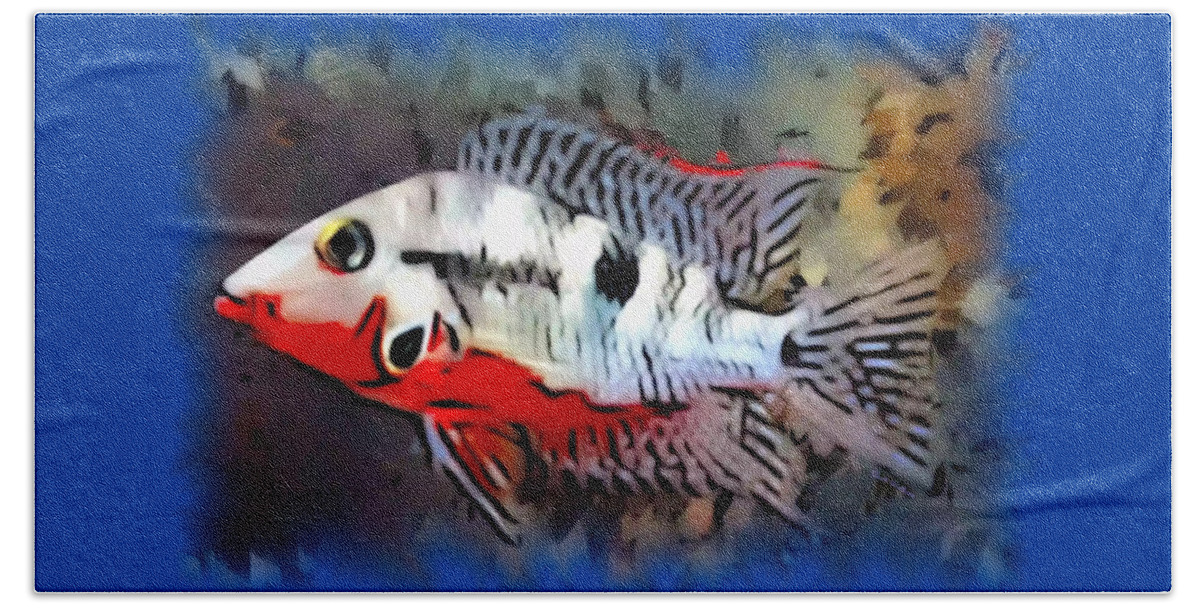The image depicts a piece of art featuring a fish swimming from right to left within a rectangular frame. The predominant subject is the fish, which is primarily white around the top and has white fins embellished with black markings. The fish's underbelly displays a vivid orange hue with some black accents, transitioning into a blood-red shade near its mouth and a thin red line along the top fin. The fish has a golden eye and a blank expression.

The backdrop consists of various textured layers. The furthest layer is a pure blue color, which is partially obscured, covering around 65% by another layer that evokes the appearance of feathers with its mixture of browns, grays, and dim green shades. This middle layer contains several wrinkles, adding to the complexity and depth of the background. The entire composition is enveloped by a blue border, framing the art piece.